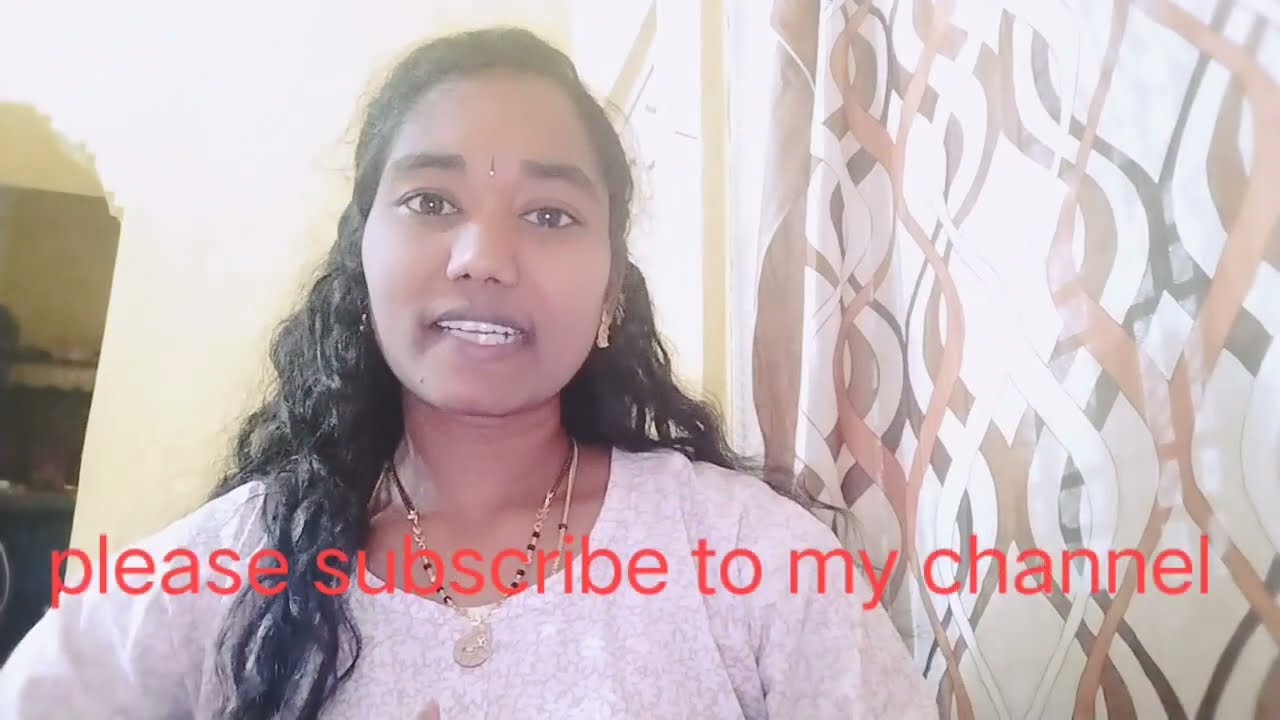In the image, we see a woman of Indian descent, looking directly at us with her mouth open, mid-speech, revealing both rows of her teeth. She has long, wavy black hair that cascades past her chest, with some strands falling over her left shoulder. A small jewel adorns the space between her eyebrows, and she is wearing gold earrings and two gold necklaces, one of which has a gold pendant. Her attire includes a patterned white and cream floral print top. The backdrop features a white curtain with curvy black lines forming vase-like shapes along with brown and white wavy patterns. To her left, there is an arched doorway leading to another room. Overlaying the bottom half of the image, in red text, is the phrase "Please subscribe to my channel."